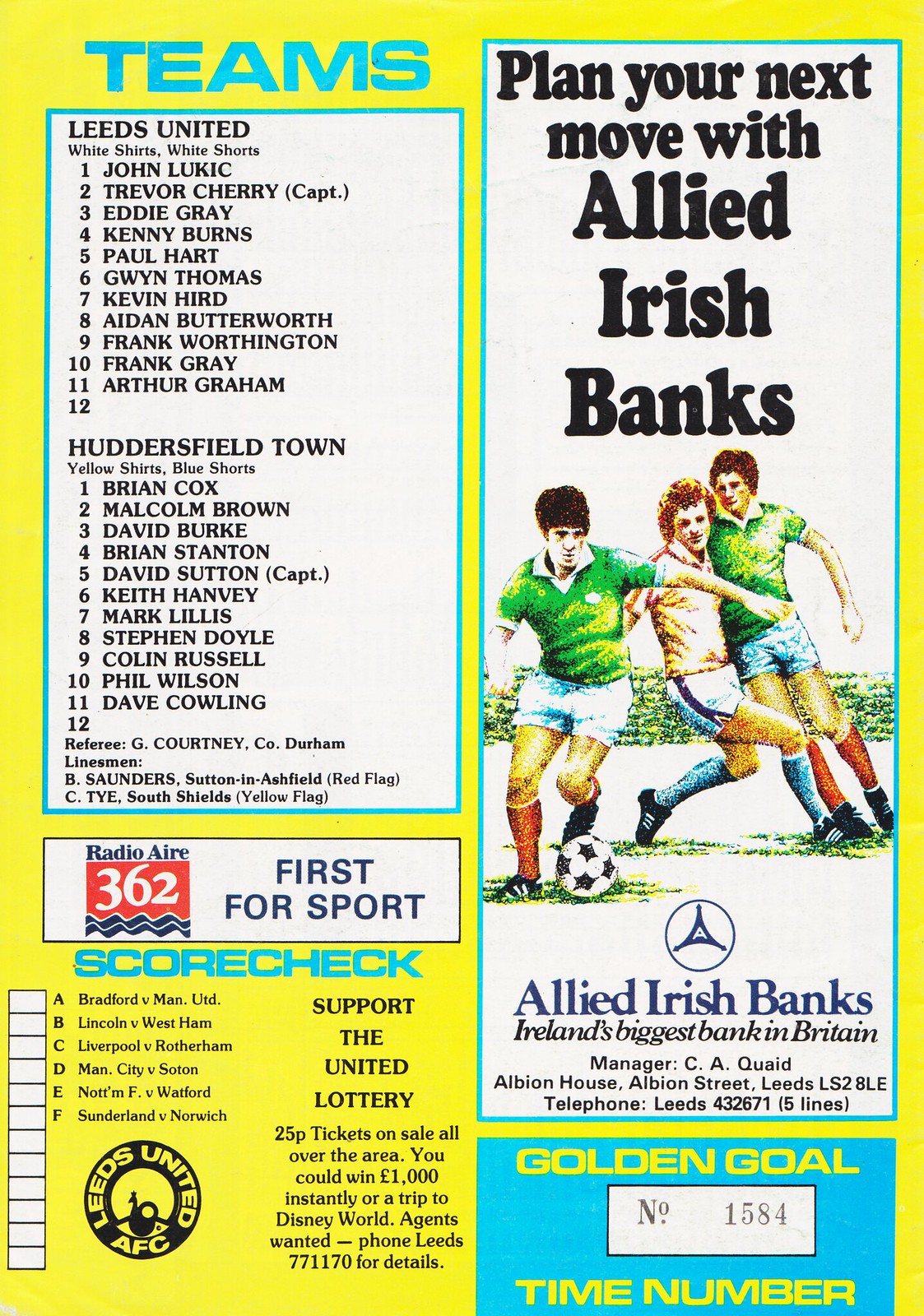This image appears to be the back cover of a yellow soccer game program or magazine. On the left side, the header reads "Teams" in blue text, followed by rosters for Leeds United and Huddersfield Town. The Leeds United roster lists players with white shirts and shorts: John Lukic, Trevor Cherry (captain), Eddie Gray, Kenny Burns, Paul Hart, Gwyn Thomas, Kevin Hird, Aidan Butterworth, Frank Worthington, Frank Gray, and Arthur Graham. Huddersfield Town’s roster, featuring players in yellow shirts and blue shorts, includes: Brian Cox, Malcolm Brown, David Burke, Brian Stanton, David Sutton (captain), Kevin Hanvey, Mark Lillis, Stephen Doyle, Colin Russell, Phil Wilson, and Dave Cowling. There are also details about the referee and linesmen. Beneath this, text reads "Radio Aire 362, First for Sport," alongside a score check area and a note to "Support the United Lottery" with 25p tickets available widely.

On the right side, a large advertisement for Allied Irish Banks showcases an illustration of three young soccer players in motion, one about to kick a ball. The ad reads "Plan your next move with Allied Irish Banks, Ireland's biggest bank in Britain," with manager C.A. Quade listed. At the bottom, there’s a small blue rectangle that reads "Golden Goal Time Number," with a white box containing the number "1584."